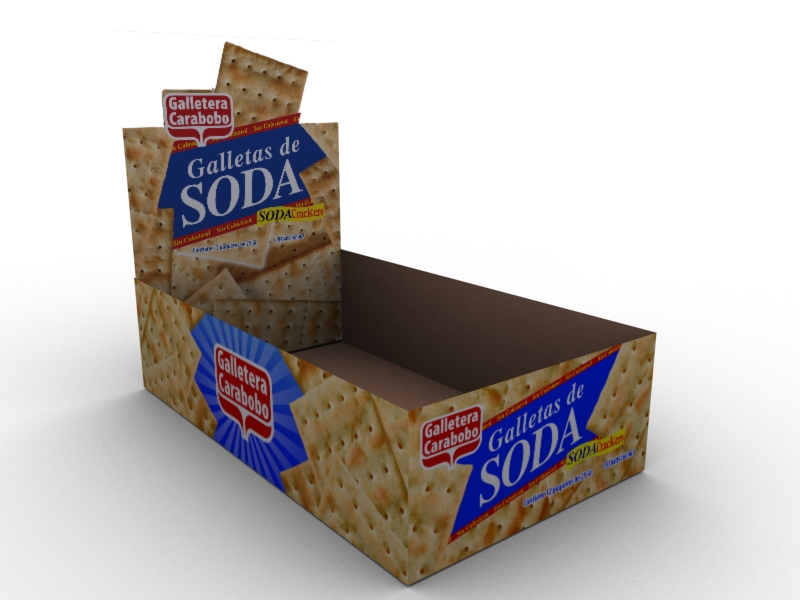The photograph showcases an empty cardboard display box, typically used in grocery stores or shops to hold soda crackers, labeled "Galletas de Soda" in both blue and yellow text. The box's outer design prominently features images of soda crackers scattered around, with consistent signage repeating the branding. The top section of the box resembles a pile of crackers with a central blue label stating "Galletas de Soda" in large white text, mirrored on the front of the box. On the left side, there's a distinctive red badge with a starlight or sunburst gradient, containing the text "Gallatera Carabobo." The background of the image is mostly white, transitioning to a very light purple on the bottom half, accentuating the detailed and vibrant display box against a softer backdrop.